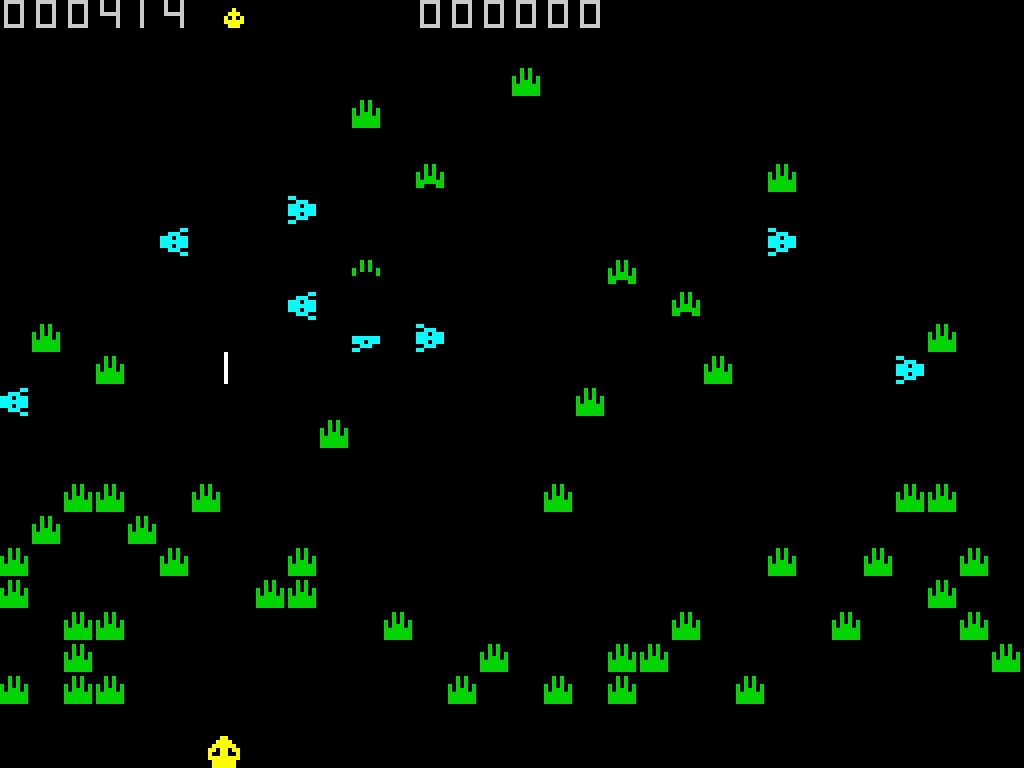This image appears to be a screenshot from a video game. At the top of the screen, there are two scores displayed. One score reads "000414" while the other shows "000000," indicating that the second player may not have started yet. The background of the screen is entirely black, creating a stark contrast with the vibrant elements in the forefront. Scattered across the screen are fluorescent shapes that resemble hands, though they lack the detailed structure of five fingers. Interspersed with these hand-like figures are a few unique face-like icons, adding variety to the visual elements.

The glowing items on the screen are rendered in bright green and light aqua colors, making them stand out sharply against the dark background. It appears that the players in the game are represented by a yellow symbol positioned on the board, highlighting their presence in the game space. The overall scene combines these elements to create a visually engaging and dynamic gaming interface.